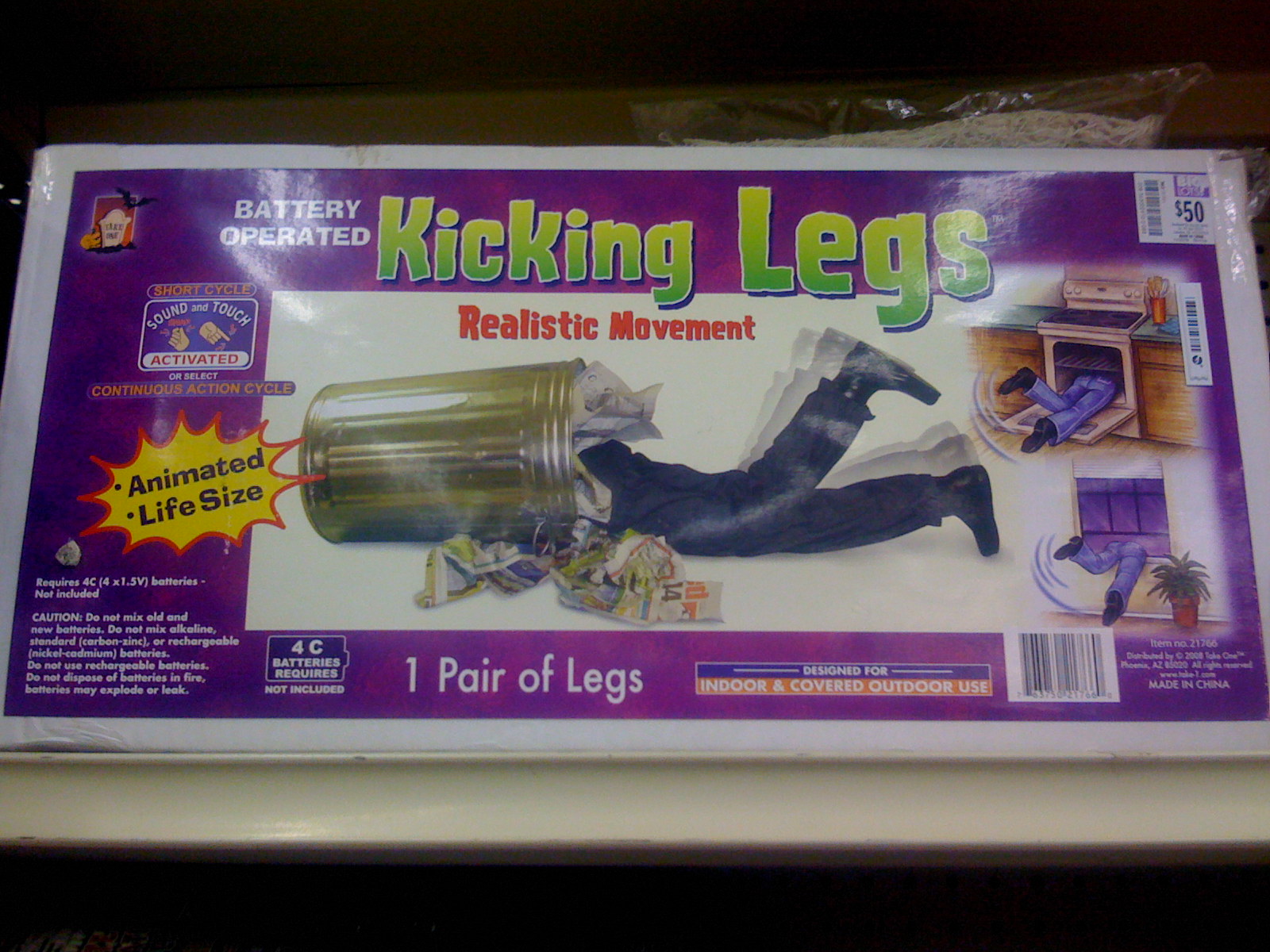The image showcases a promotional display for a quirky product called "Battery-Operated Kicking Legs." The banner, which appears to be a large billboard or label with a white border and purple background, features various informative and eye-catching elements. Dominating the top center in bold, creative green font is the product's name: "Kicking Legs," followed by the tagline "Realistic Movement." 

The central illustration captures a humorous scene: a garbage can tipped over with a pair of animated legs kicking out, as if someone is stuck inside struggling to get out. Scattered around the trash can are wrinkled newspapers, adding to the chaotic effect. 

The banner also includes a yellow starburst icon on the left, stating "Animated Life-Size" in large black font. Adjacent to this, in smaller text boxes, phrases like "Short Cycle Sound & Touch Activated" and "Or Select Continuous Action Cycles" explain the product’s functionalities. Below, a caution note details the battery requirements and user warnings.

On the right side, additional illustrations show the legs in different amusing scenarios, such as propped against a window and inside an oven, enhancing the whimsical appeal of the product. The top right corner features a $50 price tag from Big Lots, and a barcode. 

Further text at the bottom of the banner reads "One Pair of Legs" and includes more technical details like battery specifications, usage guidelines, and distributor information, indicating this product is both an oddity and a novelty item designed for indoor and covered outdoor use. The product is marketed with quirky, animated visuals to appeal to those looking for a fun and unusual decor piece.